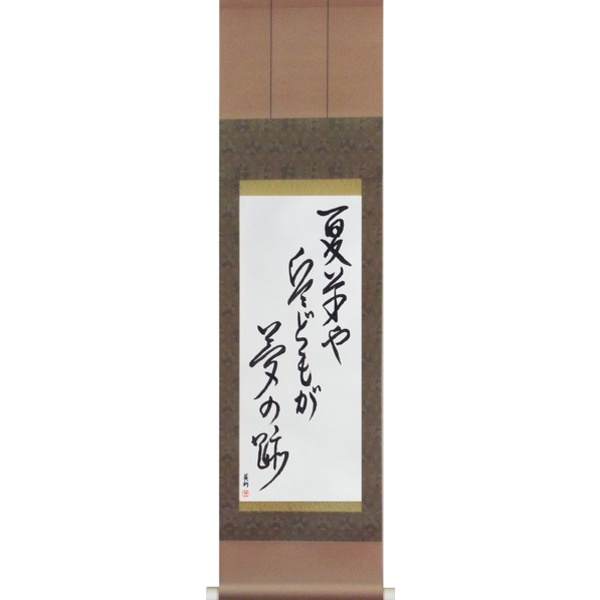This image features a large vertical scroll set against a background of light brown and dark brown shades. The darker central area showcases a white piece of paper bordered with gold at the top and bottom. The paper contains three rows of black symbols, which appear to be written in an East Asian language, possibly Japanese, Chinese, or Taiwanese. The script, resembling traditional calligraphy, is arranged from bottom to top in a vertical sequence. The scroll is framed in a brown frame and placed against a lighter brown slat wall. The detailed design highlights the traditional artistry of the scroll and its mysterious, untranslated text.